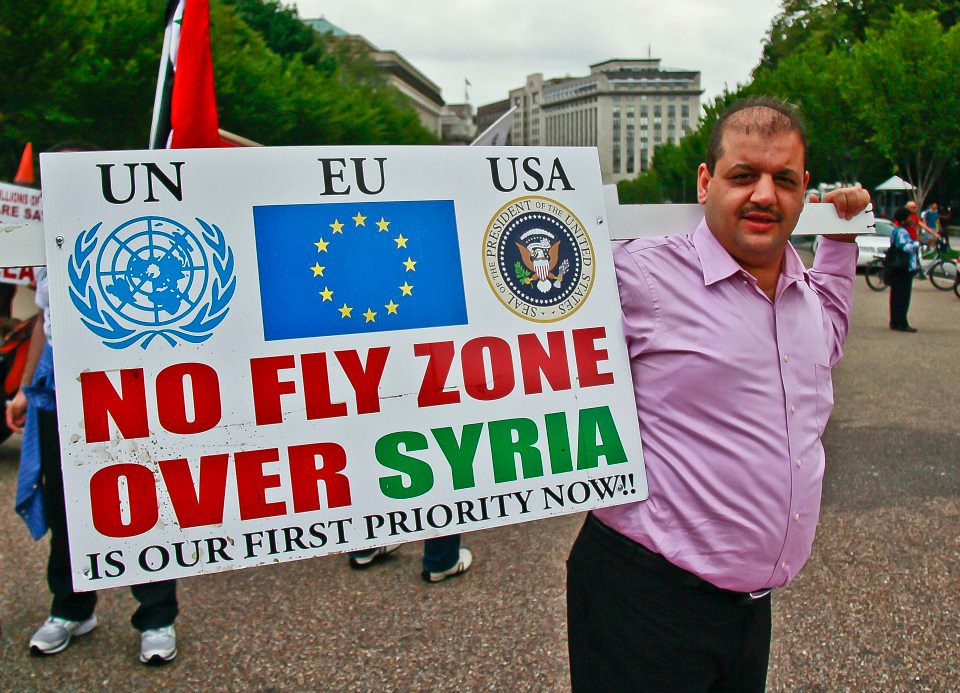In this image, a man, who appears to be Eastern European, is captured standing outside in a bustling square, seemingly engaged in a protest. He is dressed in a pink button-up shirt and black pants, held up by a belt, and looks directly at the camera while supporting a large, white wooden sign over his shoulders. The sign is prominently displayed and features the logos for the United Nations, the European Union, and the United States of America across the top, along with the acronyms 'UNU' and 'USA.' Below the logos, bold red text states "No-Fly Zone Over," followed by "Syria" in green text, and "Is Our First Priority Now!!" in black text with two exclamation points.

In the background, there are various people walking, biking, and holding their own signs, indicating a wider protest atmosphere. A white car is visible, along with green bushes and a landscape decorated with pebbles or small rocks. Additionally, the setting includes a large Capitol-style building and trees at a distance, helping to frame the scene of civic engagement and public demonstration.